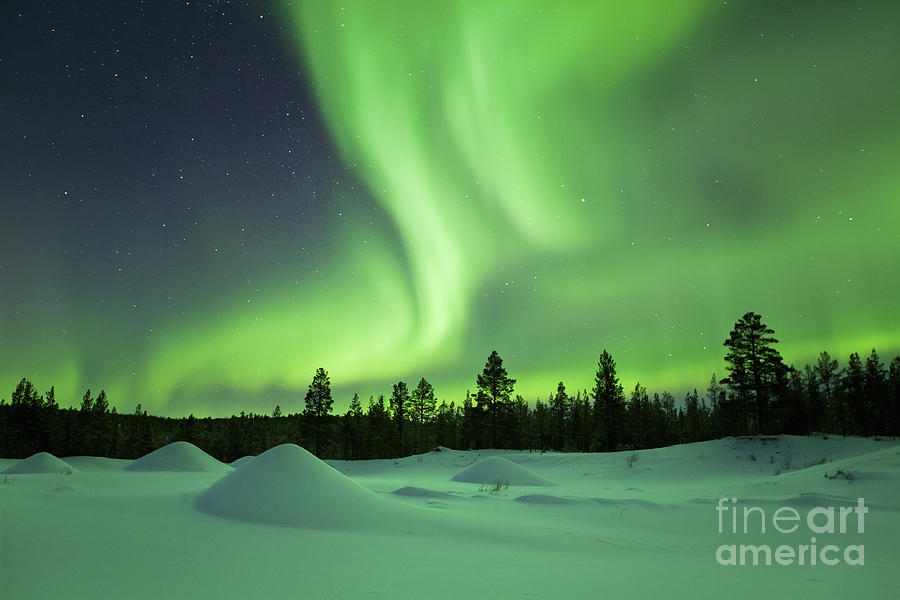A highly detailed and photorealistic drawing presents an awe-inspiring scene of the Aurora Borealis. Dominating the background, the sky splits into a hypnotic dance of green swirly lights intermingling with a dark blue to black canopy speckled with white stars. Below, the snowy ground is subtly tinged with bluish and greenish hues, adding a mystical aura to the landscape. Mounds of snow are scattered across the terrain, leading the eye to the horizon where a relatively flat, yet vibrant green landmass stretches forward. This land gives rise to dark green evergreen trees that stand tall and dense, creating a stark contrast against the illuminated sky. The entire atmosphere suggests a frigid, northern region, possibly somewhere like Canada. The image carries an ethereal quality, its overall green tint reflecting the mesmerizing light display above. In the bottom right corner, the text "Fine Art America" appears in grayish-white letters, grounding this celestial experience in the realm of artistic creation.